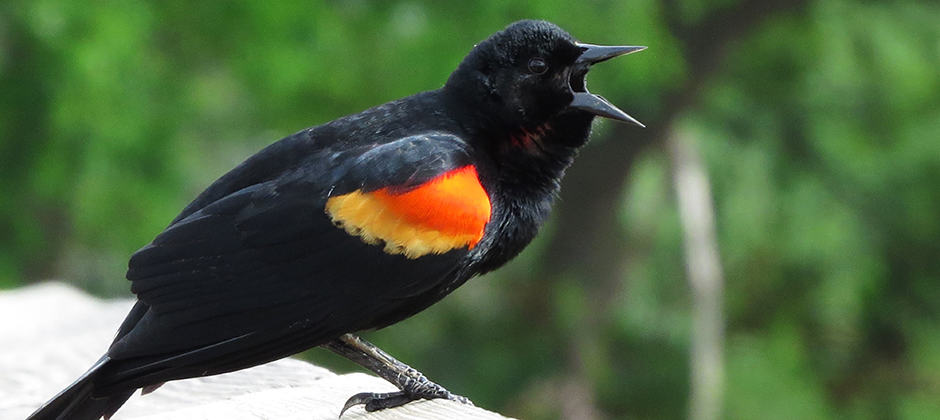This vivid color photograph captures a striking red-winged blackbird perched on a flat, white surface—possibly a fence post, stone wall, or rock—angled diagonally from the lower center to the left corner of the image. The bird is predominantly jet black, featuring a distinctly sharpened beak that's wide open, as if singing or calling. Its eyes appear small and beady. The bird's right profile is prominently displayed, with both feet clutching the edge of its perch. A stunning vivid scarlet and tangerine stripe adorns the feathers just under its right wing, creating a striking contrast with its black plumage. In the blurred background, green leaves and grayish-brown tree trunks underscore the bird's vivid coloration, ensuring your attention remains fixed on the bird’s dynamic presence. The bright epaulettes (feather patches) appear more orange than red in the sunlight, enhancing the overall vibrancy and humor of the photograph.